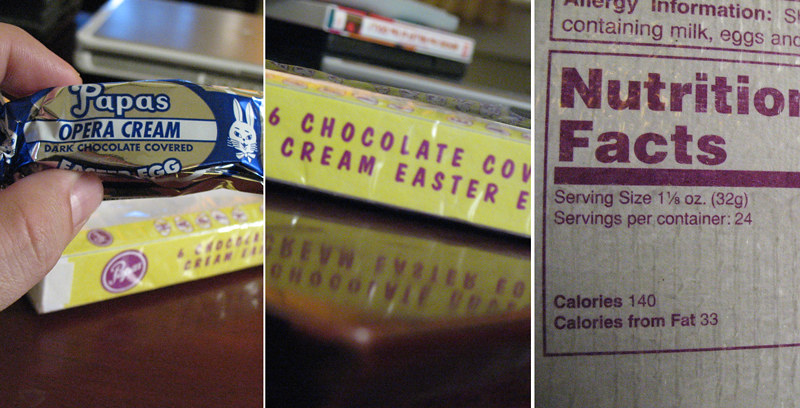The image is a horizontal, landscape-oriented composition consisting of three related photographs. On the left, a hand holds a candy wrapped in a gold and blue foil with a white label outlined in blue, reading "Papa's Opera Cream Dark Chocolate Covered." The middle photograph shows a yellow box labeled "Six Chocolate Cream Easter Eggs," written in a dark red color, sitting on a wooden table. The right image contains a zoomed-in view of the nutrition facts label, which is dark red text on a white background. The label provides allergy information: "Contains milk, eggs," and lists nutritional details including a serving size of 1 1⁄8 oz (32g), servings per container (24), 140 calories, and 33 calories from fat.